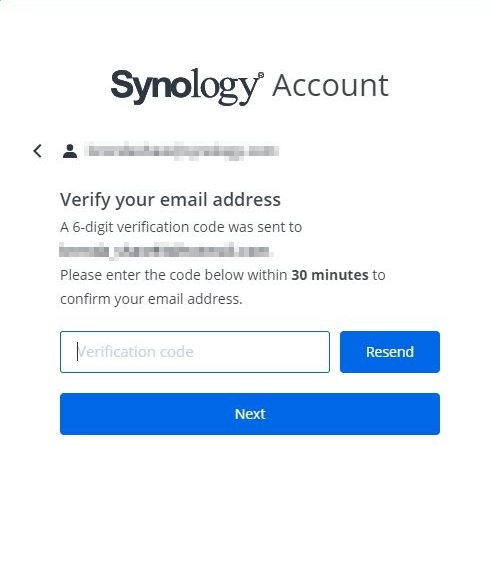This image is a low-quality screenshot, somewhat blurry and lacking sharp definition. It depicts a pop-up menu related to a Synology TM account. At the top of the menu, "Synology TM Account" is displayed in bold black font. Directly below this, there is a left-pointing arrow and a black human silhouette icon alongside a blurred-out screen name. Beneath this blurred-out section, in bold black font, it reads "Verify Your Email Address." 

The text continues to explain that a six-digit verification code has been sent to a blurred-out email address. Users are instructed to enter the code within 30 minutes to confirm their email address. Below this instruction, there is a white rectangular input field with the placeholder text "Verification Code" in gray font, and a black cursor positioned in front of the "V" in "Verification." To the right of this input field, there's a blue rectangle with "Resend" written in white font. At the very bottom of the pop-up menu, there is a long blue rectangle featuring the word "Next" centered within it.